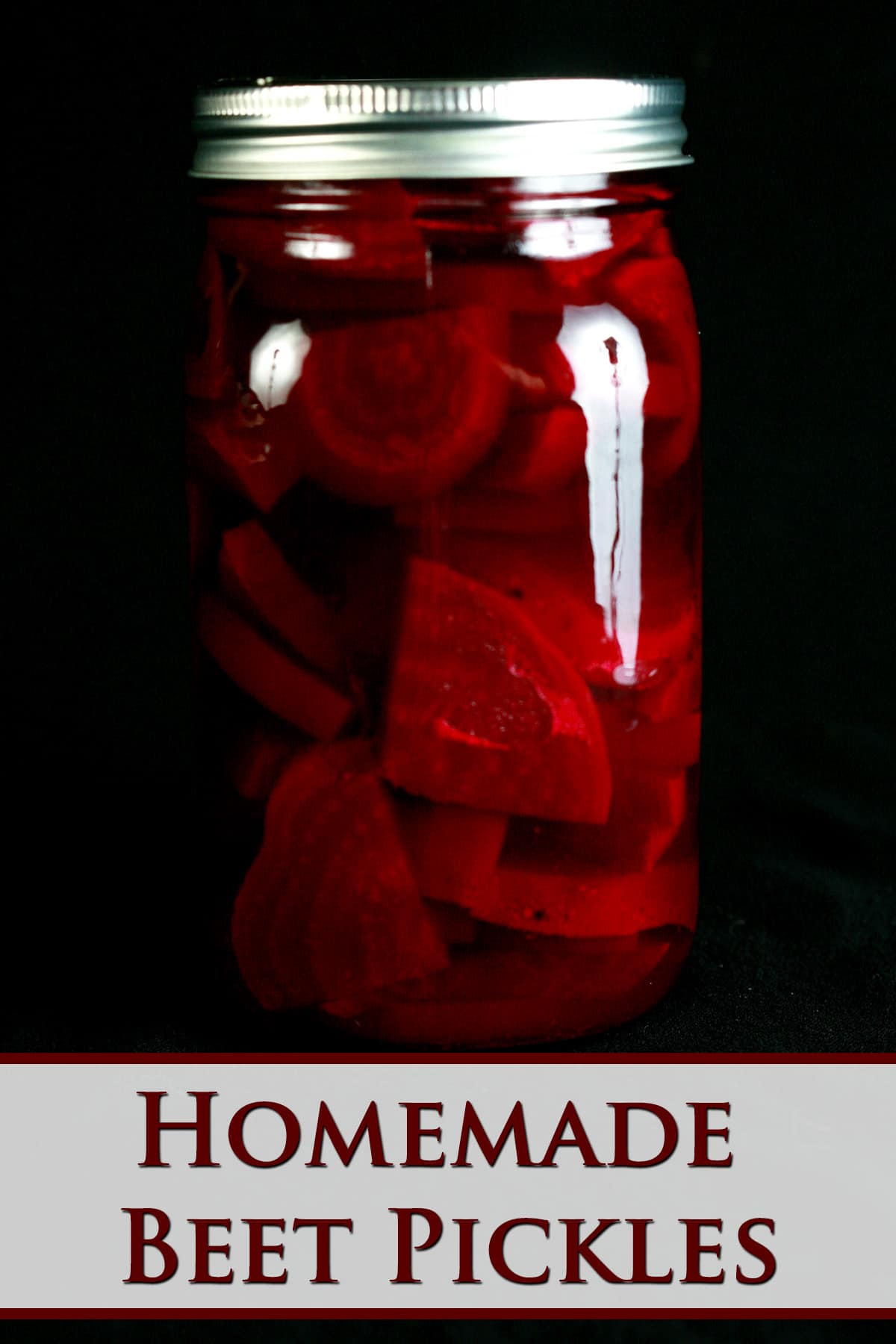The image showcases a dramatic and visually striking mason jar filled with homemade pickled beets. The jar, clear with a silver lid, stands out starkly against an all-black background, highlighted by a white light that accentuates the glossy, reddish-brown hues of the liquid inside. The jar contains neatly sliced, triangle-shaped beet pieces immersed in a pickling brine that takes on the deep red color of the beets. The bottom of the image features a gray strip with "HOMEMADE BEET PICKLES" written in bold, uppercase red letters, framed by a thin black border beneath it. The overall presentation makes it look like a well-styled photograph from a cookbook, emphasizing the homemade and preserved nature of the pickled beets.